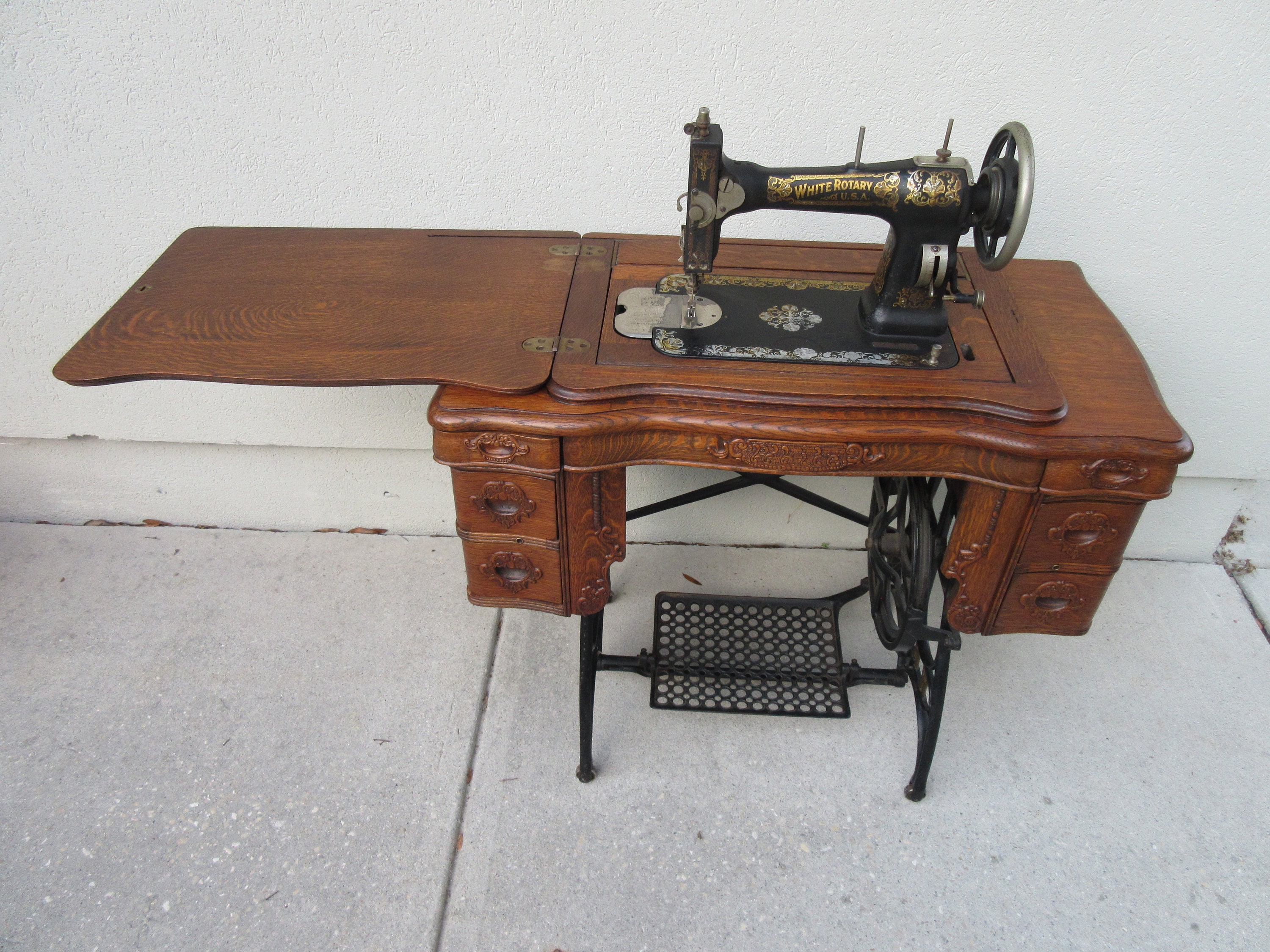This is a detailed photograph of a vintage "White Rotary" black sewing machine, built into a medium brown, ornately designed wooden cabinet. Likely originating from the early to mid-20th century, this elegant piece is a fascinating example of antique machinery. The cabinet features an extended panel and four small drawers, perfect for storing sewing supplies such as threads and scissors. Notably, the machine flaunts exquisite gold lettering and designs that read "White Rotary USA."

The sewing machine, currently lifted out of the fold-down compartment in its cabinet, showcases a remarkable blend of decorative and functional craftsmanship. The pedal mechanism, situated at the bottom of the cabinet, is composed of black metal elements, including a wheel and a small shelf or basket. This treadle mechanism, operated by foot, powers the machine, causing the needle to move up and down.

Despite its age, this sewing machine and cabinet appear to be in fairly good condition, adding to its charm and appeal. The photograph intriguingly places this classic piece outdoors on a concrete sidewalk against a white wall, which contrasts sharply with the antique's classic, detailed design. This stunning sewing machine is not just a functional appliance but also a cherished piece of historical architecture, highly desirable to vintage enthusiasts.